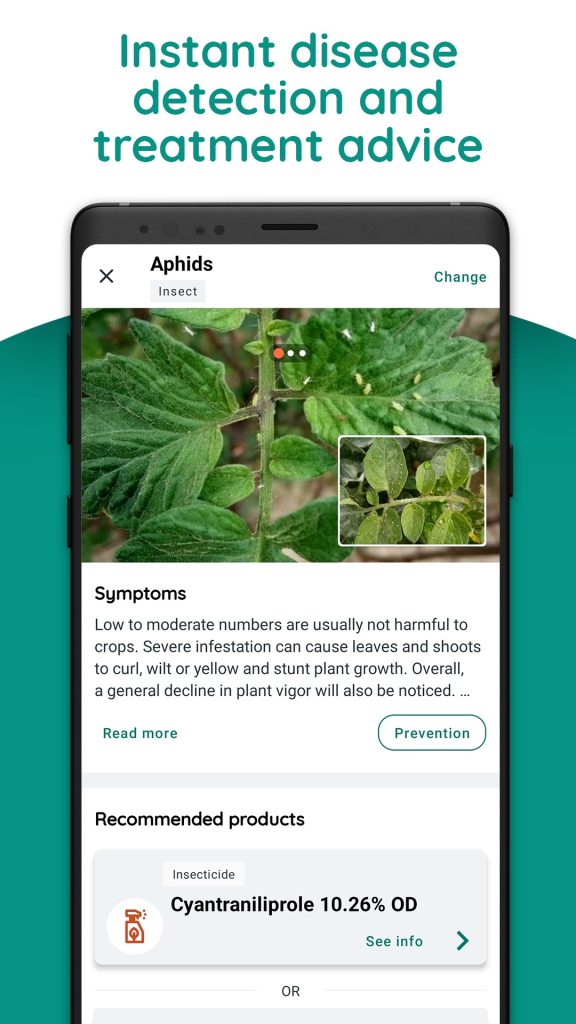In the image, a smartphone is prominently featured with its screen displaying an app for instant disease detection and treatment advice. At the top center of the image, "Instant Disease Detection and Treatment Advice" is written in greenish text. 

The smartphone itself is positioned centrally, with four camera lenses visible at the top left on the back of the phone. In the top middle of the phone's screen, there is a black rectangular bar. Directly below this, the app interface is visible. The top left corner of the screen shows a small "X" symbol. To its right, "Aphids" is displayed in bold black text. Beneath the word "Aphids," there is a small gray box containing the word "Insect." An empty space leads to the far right side of the screen, where the word "Change" appears in green text.

Below this section, the app displays a large photograph of a plant, and in the bottom right corner of this photo, there is a smaller, close-up image of the plant. Underneath these images, the word "Symptoms" is centered. Below "Symptoms," there is a paragraph explaining the impact of aphids: "Low to moderate numbers are usually not harmful to crops. Severe infestation can cause leaves and shoots to curl, wilt, or yellow, and stunt plant growth. Overall, a general decline in plant vigor will also be noticed."

At the very bottom of the image, the app indicates a section for "Recommended Products."